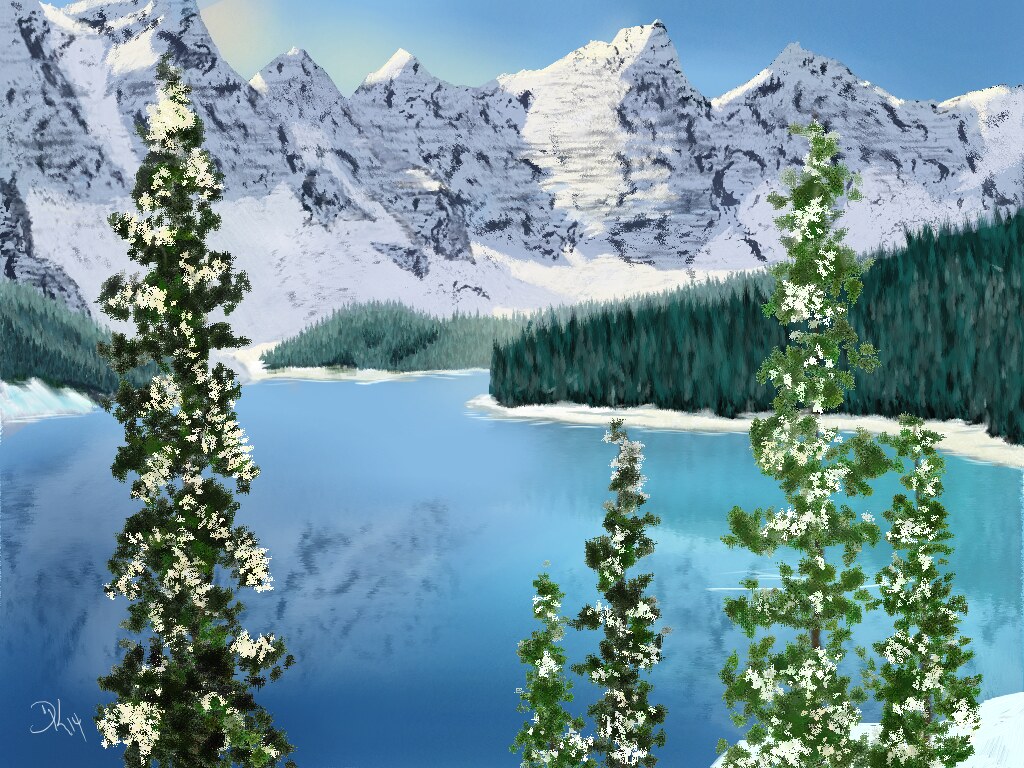This image appears to be a digital painting depicting a serene, winter landscape featuring a large, crystal-blue lake surrounded by a mix of sparse and dense pine trees. In the foreground, tall, slender pine trees are dusted with snow, their sparse leaves topped with a thin layer of ice. The lake dominates the center of the composition, its bright blue and turquoise waters vividly contrasting with the snowy surroundings. Reflecting the towering mountains and trees along its shoreline, the lake adds depth and realism to the scene. The background is graced with snow-covered mountains, their dark gray rocks peeking through the white blanket, and bathed in soft sunlight that accentuates the snow. The sky above is clear and bright blue, with a single wispy cloud or a streak of sunlight on the left side, suggesting a clear afternoon. The shoreline around the lake is densely populated with dark green pine forests without snow, adding a rich texture to the composition.